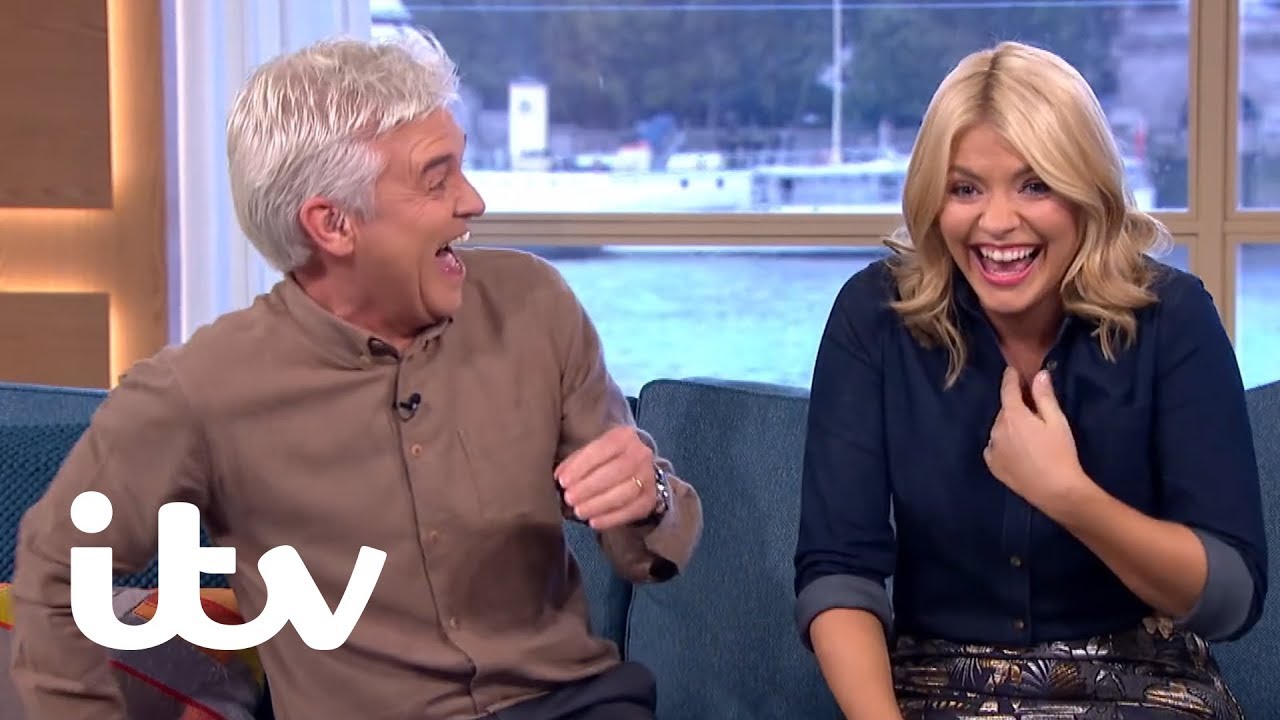In a lively scene from ITV's "Good Morning Britain," two co-hosts are captured mid-laugh. On the left, the male anchor, characterized by his completely white hair, is wearing a light brown, tan-colored button-up shirt with a portable microphone clipped to it, and a silver watch on his left arm. He is seated on a blue fabric couch, his right hand gesturing towards his chest in amusement. To his right, the female anchor with shoulder-length blonde, wavy hair, is also laughing with her mouth open, wearing a blue denim button-up shirt with the cuffs rolled up, paired with a black patterned skirt. Both are visibly enjoying a humorous moment. Behind them, through a window, an outdoor scene unfolds, likely a harbor, with water, a boat, and distant greenery. The photograph, in landscape format and full color, gives an impression of warmth and cheerful camaraderie, emblematic of a light-hearted morning television show.